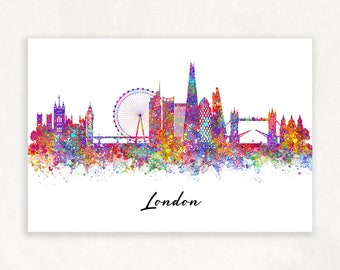This vibrant illustration of the London skyline showcases iconic landmarks such as the famous Ferris wheel, likely the London Eye, and a bridge which might be the Tower Bridge. Set on a white canvas mounted on an off-white wall, the painting prominently features the word "London" in bold black cursive letters at the bottom. The skyline, painted across the center, is rendered in an array of bright, beautiful colors including yellow, blue, purple, red, and green. The intricate design transitions from solid vibrant forms at the top to a series of colorful dots as it moves downwards, creating a striking and captivating effect. This piece, designed to attract tourists, highlights not only the historic architecture of London but also the dynamic and lively essence of the city through its dazzling color palette.